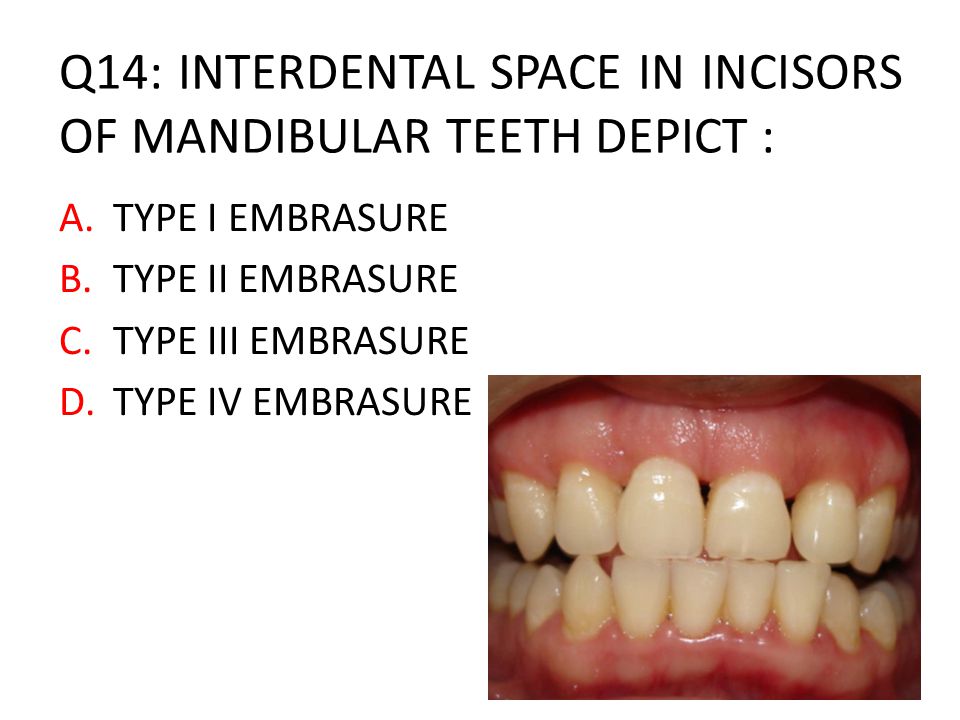In the image, there's a detailed dental photo occupying the bottom right-hand corner, prominently showcasing a close-up view of someone's teeth and gums. The person's lips are retracted, revealing both the upper and lower rows of teeth and the pink gums. The teeth have a slight yellowish tint, and the overall appearance is somewhat unsettling due to the exposed view. In the upper left-hand corner, taking up about half of the image space, there's a significant amount of black text on a white background. The text reads: "Q14: interdental space in incisors of mandibular teeth depict," followed by options in red text labeled A, B, C, and D. These options specify different types of embrasures: "A) type I embrasure," "B) type II embrasure," "C) type III embrasure," and "D) type IV embrasure." The numbers one through four are presented in Roman numerals. This appears to be a quiz question, likely intended for dental students to identify the correct type of embrasure based on the dental photo provided.